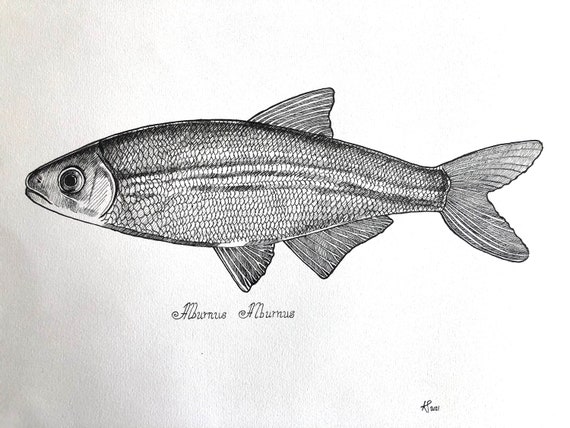This is a black and white, highly detailed drawing of a fish depicted in profile, sketched in pencil on a light gray, paper. The fish, identified as "Alburnus alburnus," commonly known as the bleak fish, has very pronounced lateral lines, extending from its gills to its tail. The fish has a large, black, and perplexed-looking eye, with the intricate scales meticulously detailed, adding texture and depth. The dorsal and tail fins, as well as the two bottom fins – one triangular and the other almost rectangular – are finely lined, giving a sense of their texture and movement. The genus and species names, written in Latin, are in fine print below the fish. The scales and the stripes running the length of the body, ending at the tail, enhance its realistic portrayal. The artist's barely discernible signature appears in the lower right-hand corner.